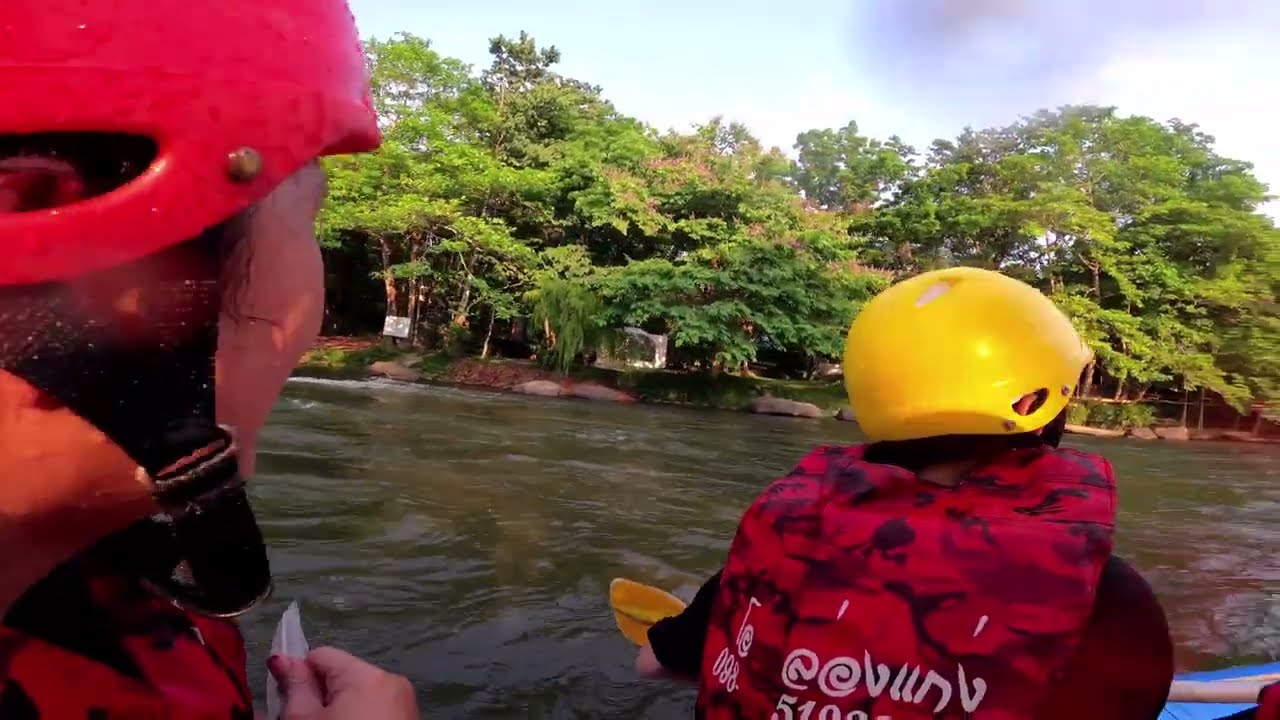The photograph portrays two people kayaking on a river or lake, captured from behind. The person on the left, closer to the camera, is wearing a red helmet and has brownish hair visible beneath it. Their right arm is raised, holding either a strap or possibly the oar against their chest. The individual in front on the right side is equipped with a yellow helmet and is dressed in a red and black life vest over a black t-shirt. A yellow paddle is partially visible, with its stick extending horizontally across the lower part of the image. In the background, the shoreline is densely covered with tall trees with widespread branches and green leaves, suggesting a lush, wooded environment potentially in an Asian country. Notably, a small white sign is affixed to the leftmost tree. Both individuals appear to be of Asian descent, and the scene suggests they are navigating through calm waters surrounded by nature.